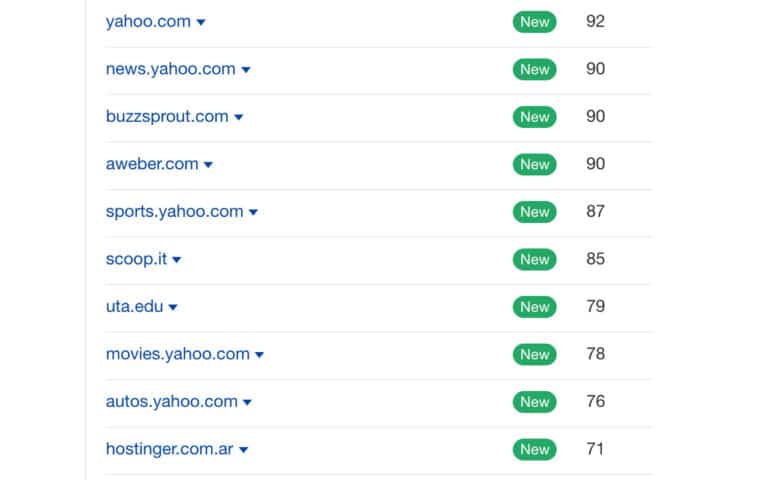The image features a clean white background highlighting a list of websites primarily aligned on the left. Each website name appears within its own row, accompanied by a blue drop-down arrow to its right. A light gray vertical line marks the boundary on the far left side of the image. 

On the right, two distinct columns display additional information: the second column from the left contains a series of green, oblong-shaped buttons labeled "New," each aligned with a corresponding website name. The third column on the far right lists a series of numbers, one per row, aligning with the respective websites. 

The websites listed from top to bottom are:
1. yahoo.com
2. news.yahoo.com
3. buzzsprout.com
4. aweber.com
5. sports.yahoo.com
6. scoop.it
7. uta.edu
8. movies.yahoo.com
9. autos.yahoo.com
10. hostinger.com.ar

Each row separating these website entries is delineated by a horizontal line, providing a clear and organized structure to the information presented.